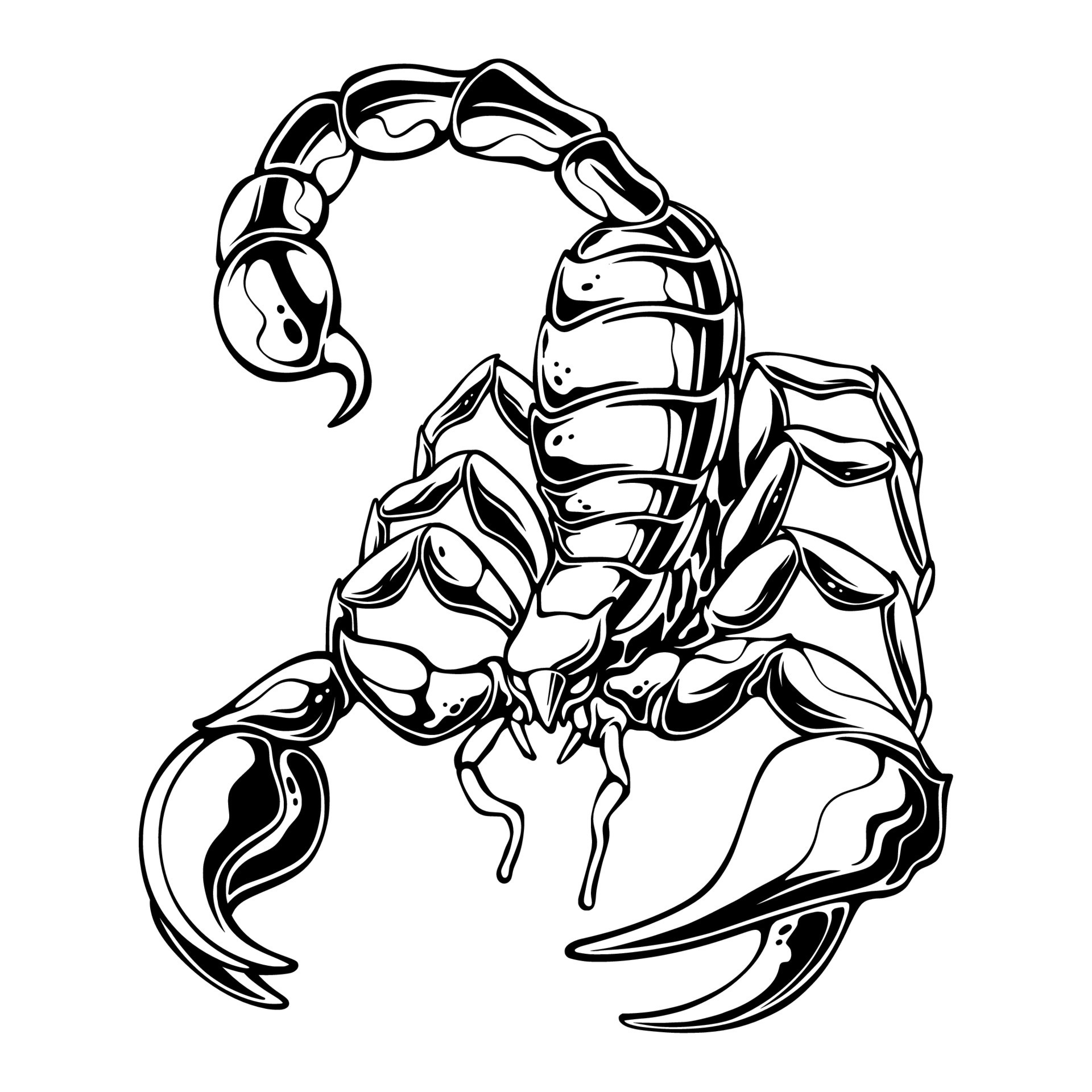This black-and-white image is a detailed, cartoon-style drawing of a scorpion. The scorpion's tail curves up and over its back, ending in a pointed stinger that leans towards the left, giving the impression it is poised to strike. The drawing features an asymmetry in the large pincers: the left pincer is more closed, larger, and more spread apart, while the right pincer is smaller, more together, and not as pointed. The scorpion's overall appearance is accentuated with many dots on its scales, giving it a textured look. The creature also has two large front antennae and six visible legs in addition to its two imposing pincers, which appear to be ready for action. The scorpion's expression appears angry, enhancing its menacing stance in this graphic representation.